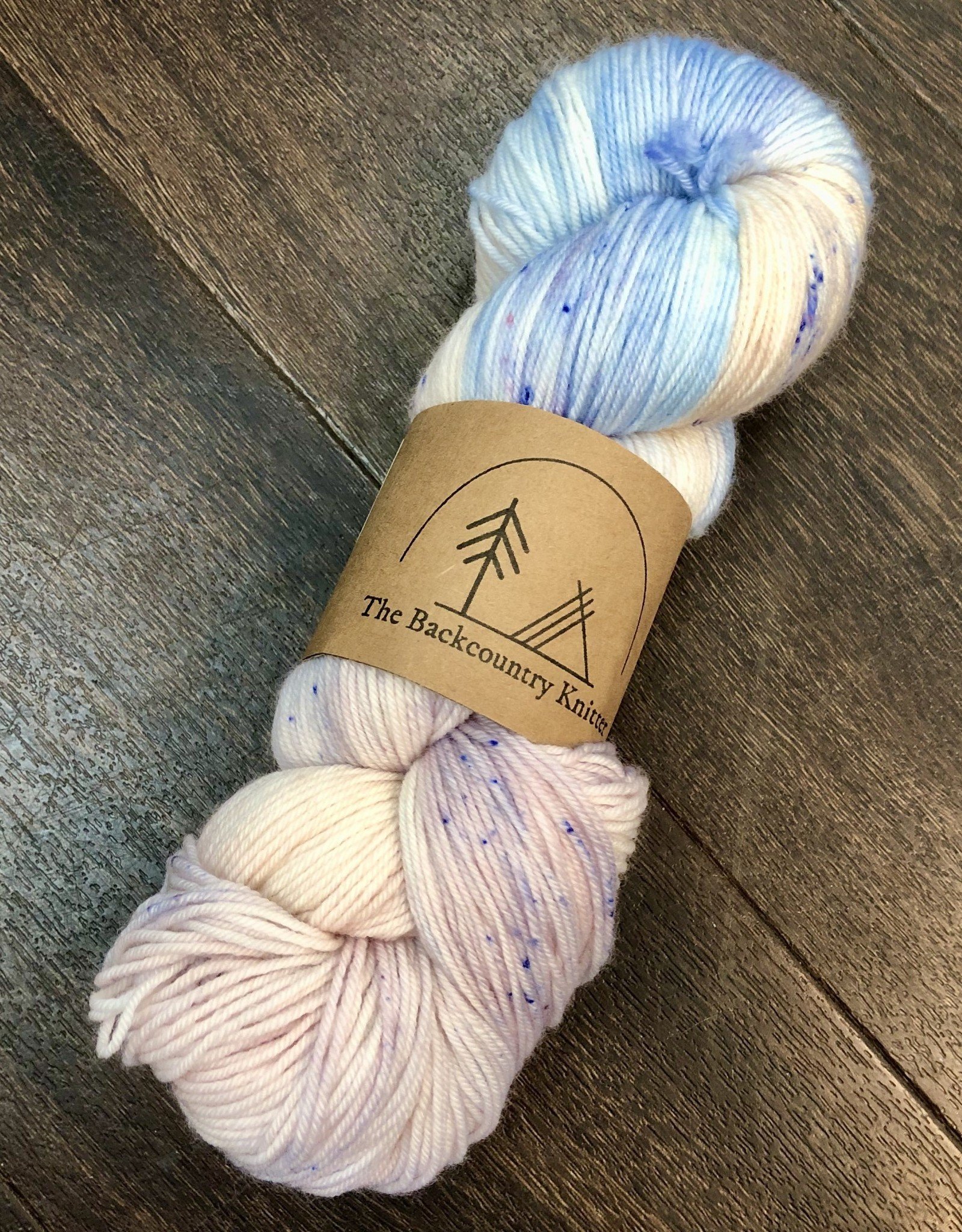In the photograph, a colorful bundle of tubular-wrapped yarn, labeled "The Back Country Knitter" on a brown paper band, lies on a clean, shiny, dark brown hardwood floor. The yarn features a primarily neutral base with splashes of blue at the top, yellow, light pink, and occasional purple spots, giving it a dyed appearance. The label showcases a tree and tent illustration above the brand name. The yarn stretches from the lower left corner to the upper right corner of the vertically oriented image.